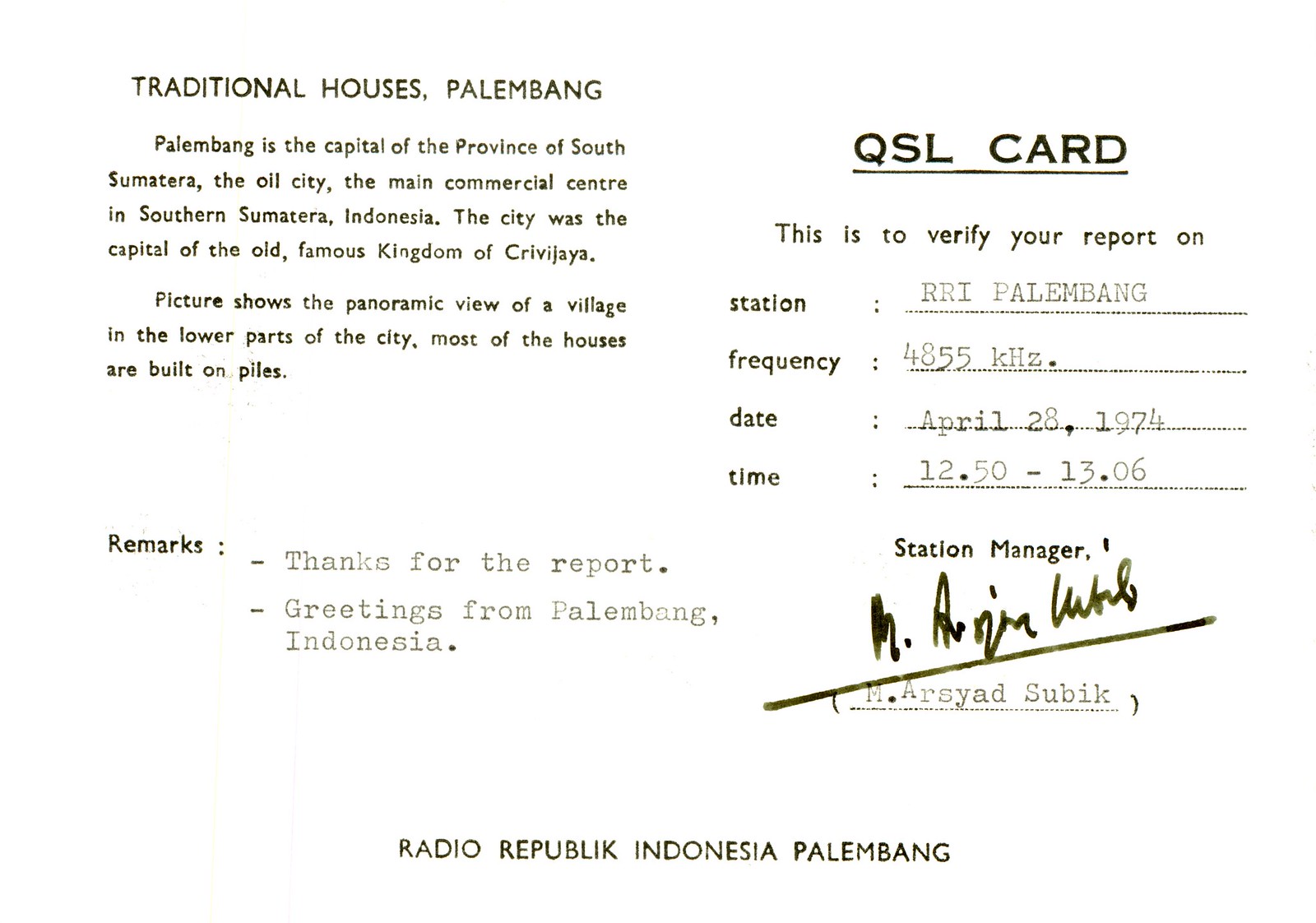The image is a scan of a QSL card, used for verifying a radio listener's report. In the upper right-hand corner, it is labeled "QSL card." It features pre-printed and typewritten elements on a white background. The main title, "Traditional Houses, Palembang," is in the upper left-hand corner. Below this, two paragraphs provide context: "Palembang is the capital of the province of South Sumatera, known as the oil city and the main commercial center in southern Sumatera, Indonesia. It was the capital of the old famous kingdom of Srivijaya." The second paragraph describes the image: "The picture shows a panoramic view of a village in the lower parts of the city, where most houses are built on piles."

The card details a specific radio report verification. It lists the station "RRI Palembang," frequency "4855 kHz," date "April 28th, 1974," and time "1250-1306." In the lower left corner, under "Remarks," it says, "Thanks for the report. Greetings from Palembang, Indonesia." At the bottom center, it states "Radio Republic Indonesia, Palembang." The station master's name, M. Aryad Subic, is typed and signed in marker. The card uses black, white, and slight shades of brown or gray, with all information clearly spaced and legible, giving it the appearance of a pre-printed postcard meant for correspondence from a radio station.